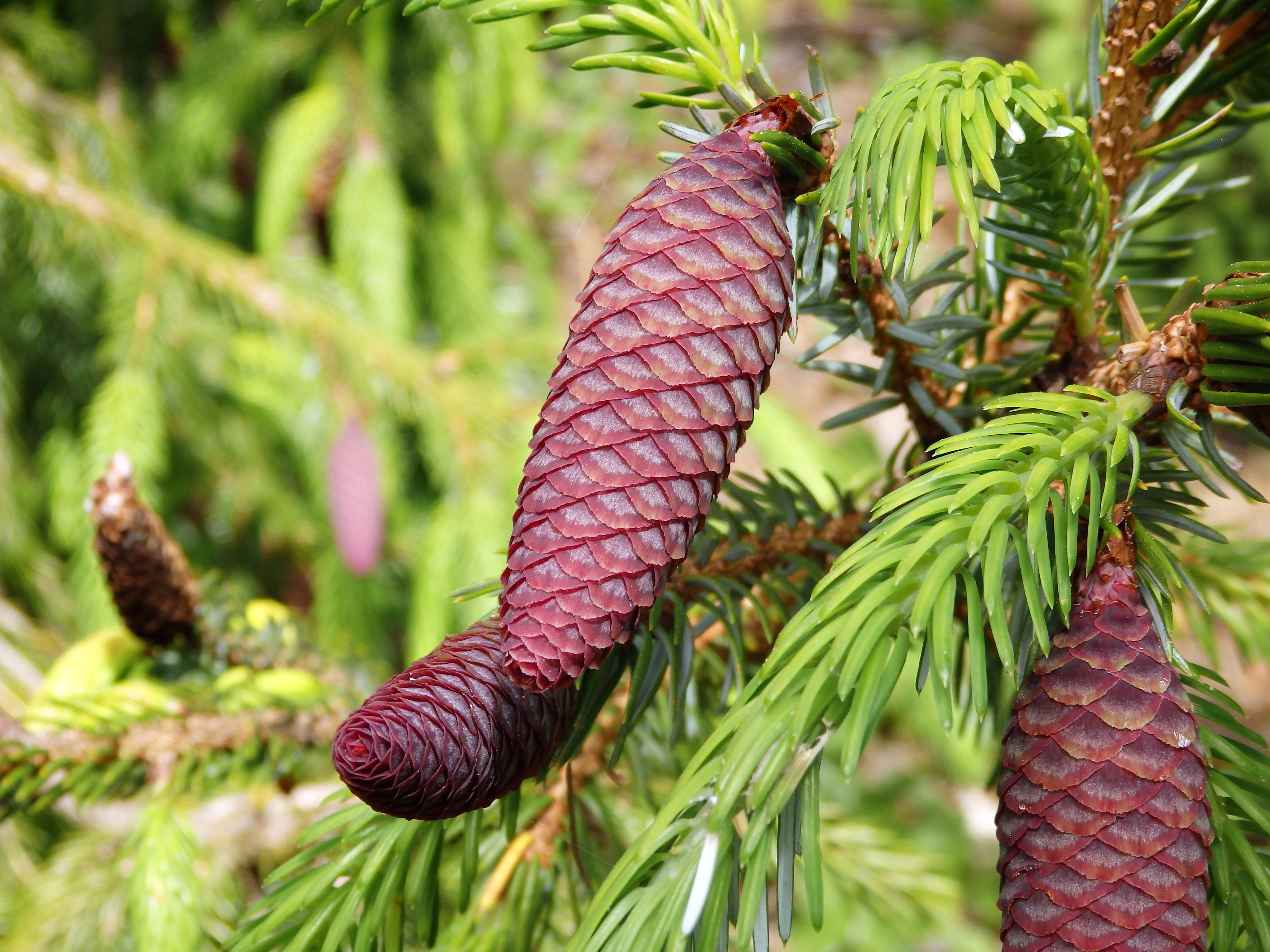This detailed color photograph, captured in bright daylight using a professional camera, showcases a vibrant and healthy pine tree branch adorned with multiple pine cones. The image is in landscape orientation and presents a close-up view with an emphasis on the natural beauty of the scene. 

The central subject is a cluster of elongated, elliptical pine cones at various stages of maturation. The most prominent cone, positioned towards the center-top of the image, appears to be in an early stage of development with its individual leaves yet to fully blossom. Surrounding this are three more cones: one partially visible beneath the central cone, a larger one on the right, and a smaller cone just below the midpoint on the left. These cones range in color from a fresh, reddish tint to the more familiar brown hue, indicating varying degrees of maturity.

The right side of the photograph is in sharp focus, clearly depicting the light green, needle-like leaves and branches, while the left side gradually transitions into a blur, creating a sense of depth and drawing the viewer's attention to the detailed subject matter. The background consists of multiple tufts of green pine leaves, further enhancing the natural, serene atmosphere of the image. There are no people, animals, or identifying landmarks present, allowing the viewer to focus solely on the intricate details of the pine cones and foliage.